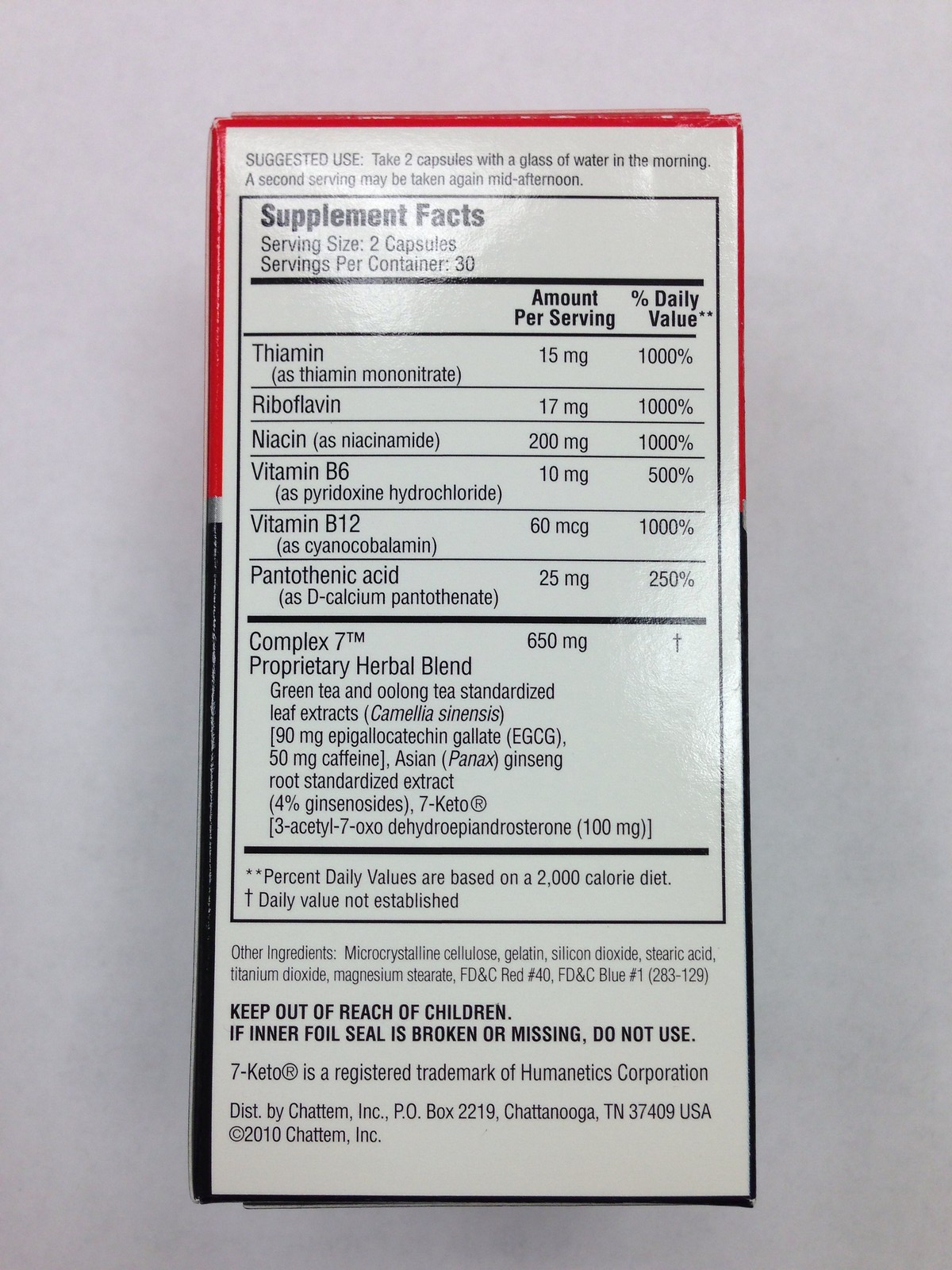The photograph captures a close-up view of a red and dark green rectangular box, situated on a white counter, displaying its nutritional label. This label, written in black text, details suggested use: two tablets with a glass of water in the morning, with an optional second serving in the mid-afternoon. The label includes serving size (two capsules) and servings per container (30). Specific nutrients listed are thiamin (15 mg, 1,000%), riboflavin (7 mg, 1,000%), niacin (200 mg, 1,000%), vitamin B6 (10 mg, 500%), vitamin B12 (60 mcg, 1,000%), pantothenic acid (25 mg, 250%), and a 650 mg blend labeled as "complex 7," which includes a proprietary herbal blend with 90 mg of standardized leaf extracts of green tea and oolong tea, containing 50 mg of caffeine, and Asian ginseng root extract. The label also includes warnings written in bold, advising to keep the product out of reach of children and not to use if the inner foil seal is broken or missing. The upper section of the label has a red border, while the lower section is outlined in black.